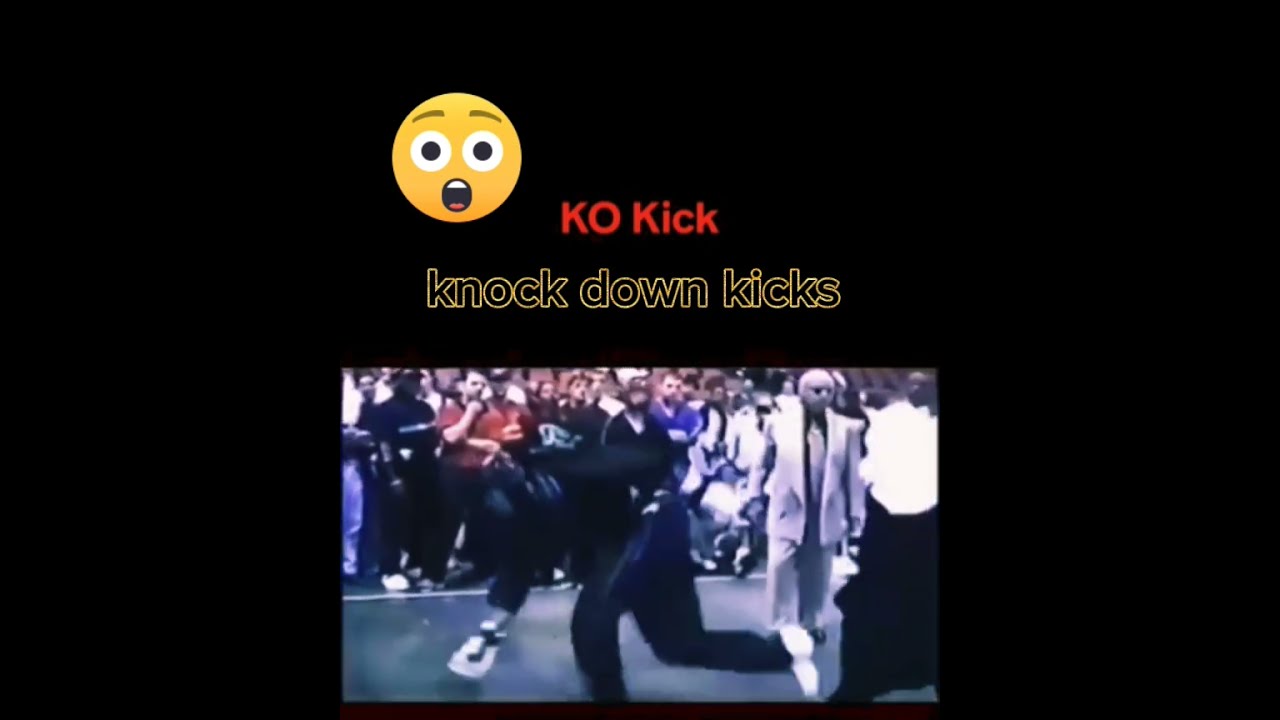The image displays a dynamic scene set against a black background, focusing on a surprising and intense moment. On the left side near the middle, a wide-eyed, open-mouthed, surprised emoji face captures immediate attention. To the right of the emoji, bold red capital letters spell out "K-O KICK." Beneath this, in letters featuring a yellow outline with a black center, the text "KNOCKDOWN KICKS" stands out.

Below the textual elements, there is a color picture depicting a sporting event. The image is slightly blurry, showing two figures in a fight, surrounded by a large audience of fans in the background. To the right of the fighters, a man dressed in a white suit with black sunglasses observes the scene. The crowd in the arena adds a palpable sense of excitement and anticipation to the scene. The overall layout suggests a lively and dramatic sporting event, possibly intended for a social media presentation, highlighted by the bold text and emotive visuals.